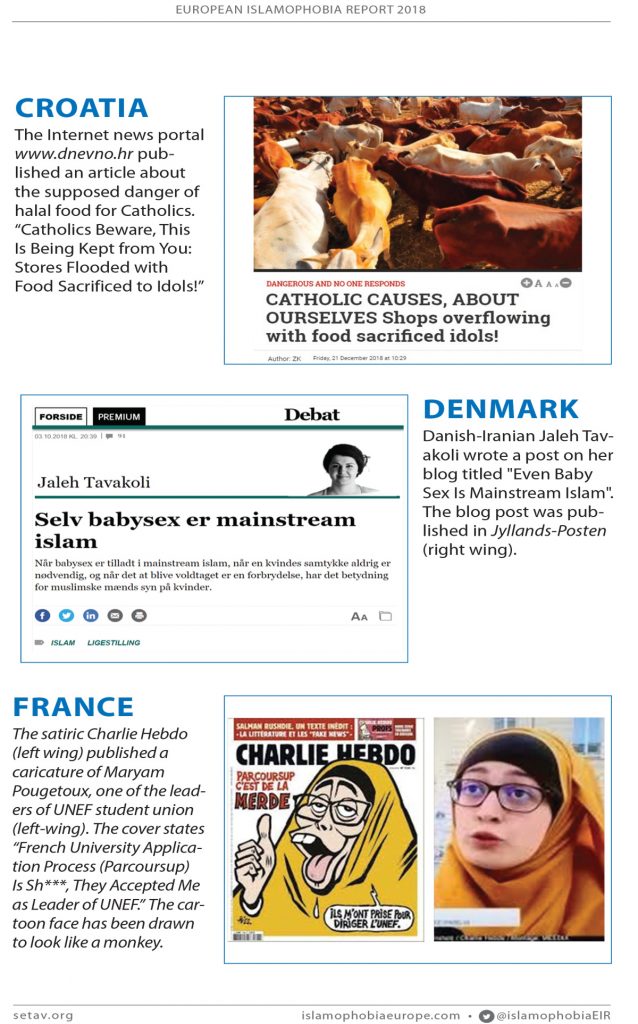The image features the "European Islamophobia Report 2018" prominently in gray at the top center, with a thin gray line beneath it. To the left and below, the word "CROATIA" is displayed in large blue capital letters. Below this title, the text in black details an article from the Croatian internet news portal dnevno.hr, which sensationalizes the dangers of halal foods for Catholics. The headline reads: "Catholics Beware: This is Being Kept from You, Stores Flooded with Food Sacrificed to Idols!"

On the right-hand side of the image, there is a photograph depicting a group of cows. Beneath the photograph, bold red text declares: "Dangerous and No One Responds! Catholic Concern: Stores Overflowed with Food Sacrificed to Idols!"

On the right side of the image, the word "DENMARK" appears in large blue capital letters. Below this, the text informs us that Danish-Iranian Jaleh Tavakoli wrote a controversial post on her blog titled "Even Baby Sex is Mainstream Islam." Published in the right-wing publication Jyllands-Posten, the blog post's provocative title is highlighted, though its exact implications are not clarified within this caption.